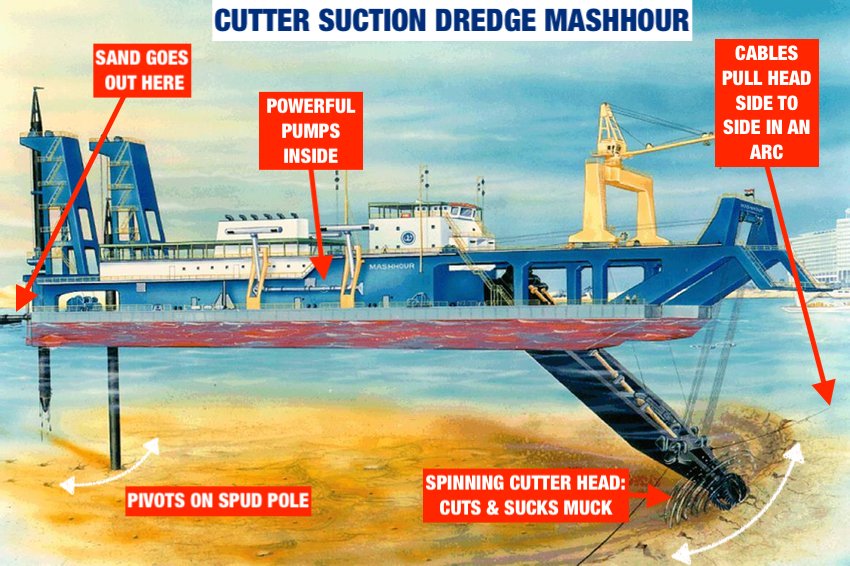This is a detailed, illustrated diagram titled "Cutter Suction Dredge Mash Hour" in blue, all-cap text set against a white rectangle at the top. The diagram features a broad, blue metal ship with a red bottom, floating on a light blue ocean. The ship is shown in cross-section to reveal its internal mechanics and interactions with the ocean floor.

The deck of the ship is populated with various structures, including a yellow crane for loading and unloading, and a white control station where the captain likely stays. The image also depicts a blue sky with white clouds in the background, and some distant white buildings with windows on the right.

The diagram includes several red boxes with arrows pointing to different parts of the ship, each with white text labels for clarity. At the back of the ship, one box labels where "sand goes here," indicating the sand collection area. Another label in the middle of the ship points to the "powerful pumps inside."

At the front, an arrow explains how "cables pull head side to side in an arc." Beneath the waterline, the ship employs a black metal "spinning cutter head" that "cuts and sucks muck" from the seabed, showing how it drills into and disturbs the brown sediment on the ocean floor. Additionally, there are stabilizing black rods referred to as "spud poles" on either side of the ship, labeled with "pivots on spud pole" and demonstrated with double-sided arrows to simulate their pivoting action.

Overall, the image conveys the complex workings of a cutter suction dredge, highlighting the ship’s components and their purposes in reclaiming sediment from the seafloor.